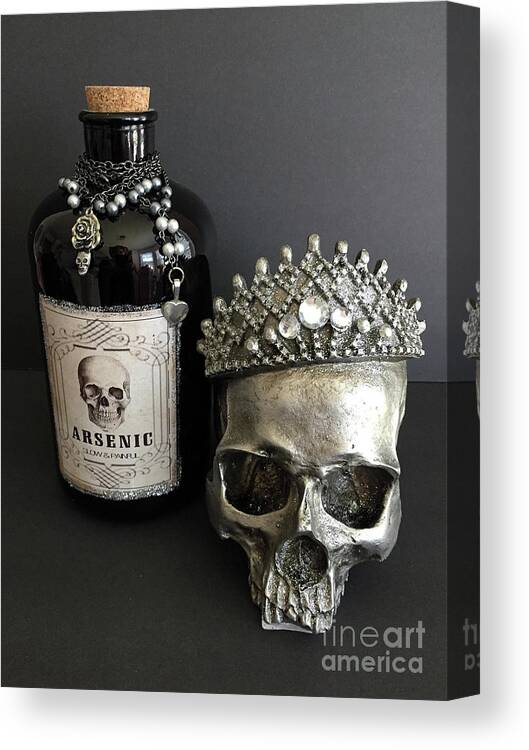This image is a detailed still life illustration printed on a wraparound canvas, likely created for advertisement or online use. The canvas features a predominantly gray background that transitions from lighter at the top to darker at the bottom. 

On the left side of the canvas, there is a black glass bottle adorned with an ornate, silver jewelry necklace, which includes a silver flower, skull, and heart among its beads. The bottle has a cork stopper and a large white label displaying a human skull with an intricate border around it. Below the skull, the label is marked with the words "arsenic" in bold, followed by the smaller text "slow and painful." The reflective surface of the bottle shows the faint reflection of a window and possibly the person taking the photograph. 

To the right of the bottle sits a silver skull sculpture without a lower jaw, its eye sockets and nasal cavity painted black to emphasize depth. It is crowned with a silver tiara adorned with rhinestones or diamonds, adding a touch of macabre elegance. 

At the bottom right corner of the canvas, the text "Fine Art America" is inscribed in light gray lowercase letters. The wraparound edges of the canvas continue the artwork, creating a seamless depiction around the sides.